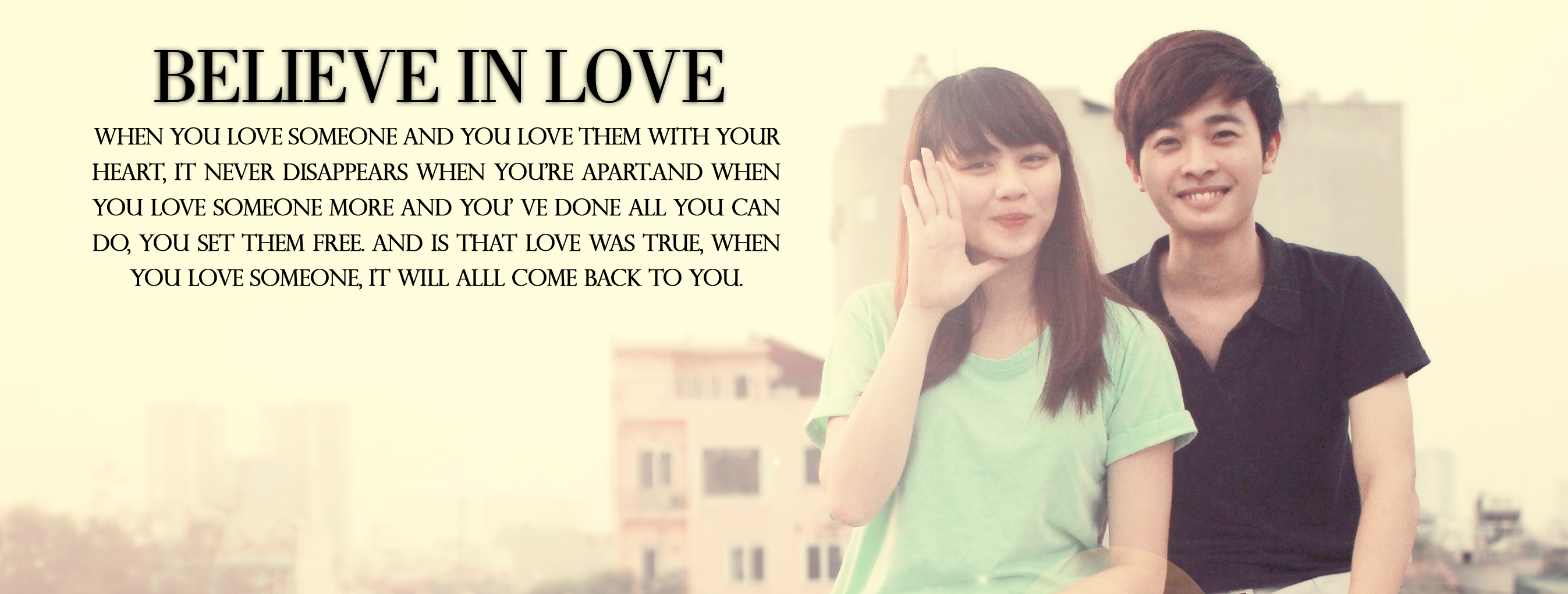The photograph captures a smiling Asian couple on the right, with the woman in a light blue T-shirt raising her hand and dark brown hair, and the man with light brown hair wearing a black collared polo shirt. They are positioned against a backdrop of multi-storied buildings, under a sky with a yellowish tint, possibly due to pollution or a filter effect. On the left side of the image, in bold black text, is an inspirational quote: "Believe in love. When you love someone and you love them with your heart, it never disappears when you're apart. And when you love someone more and you've done all you can do, you set them free. And if that love was true, when you love someone, it will all come back to you." The imagery and text together convey a romantic and uplifting theme.